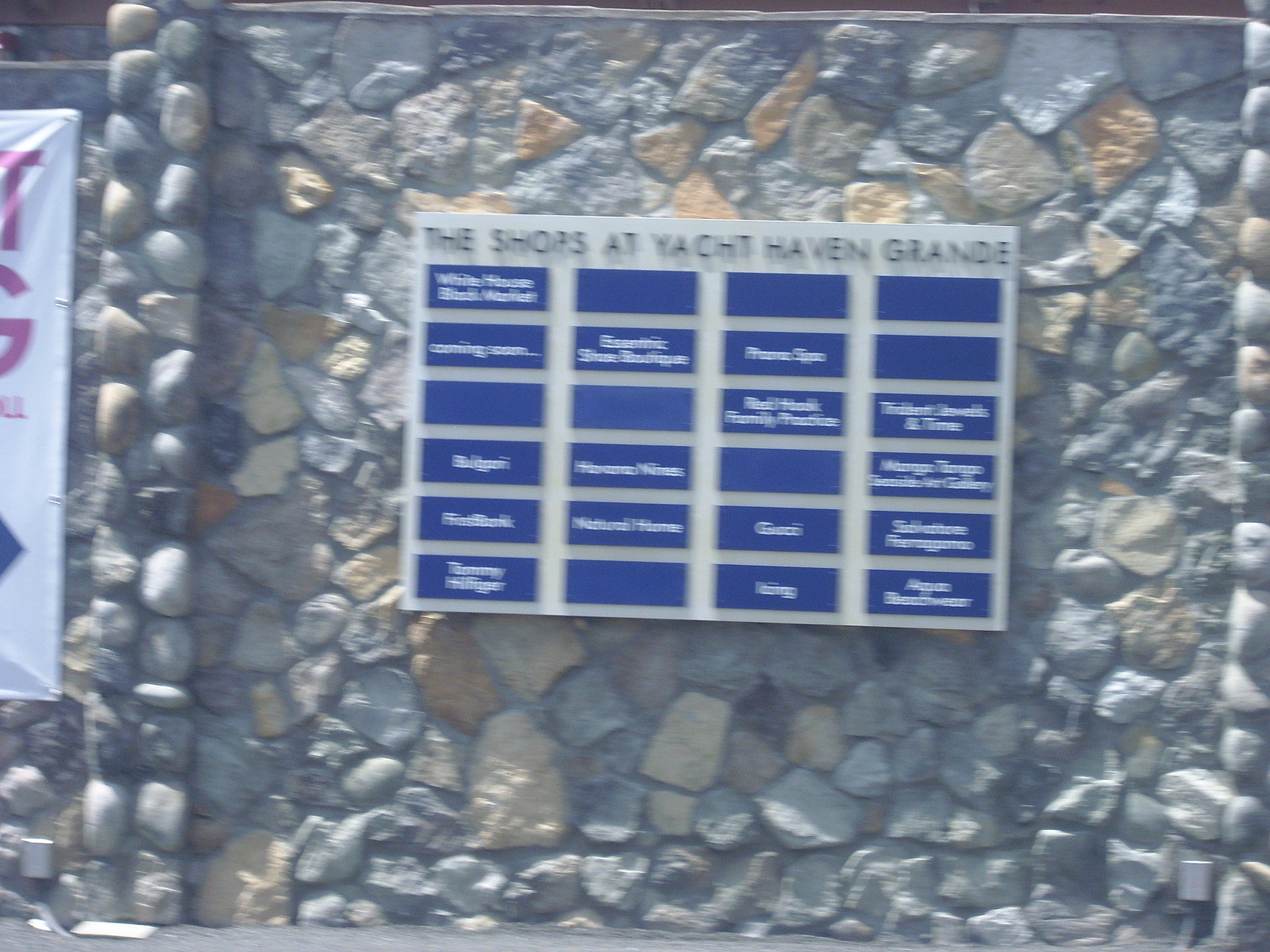This photograph captures the side of a building constructed from a variety of colored rocks, predominantly featuring hues of white, brown, and gray. The image is notably out of focus, adding a blurry effect to the scene. Centrally placed on the building's facade is a rectangular white panel that bears a black tiled inscription reading "The Shops at Yacht Haven Grande." Below this panel are four rows of blue squares, each row comprising roughly six squares. Some of these squares include white lettering, although the exact text is indiscernible due to the blurriness. To the left of the image is a partially visible white sheet with some purple text, with distinguishable letters "T" and "G," and possibly a blue letter near the bottom. The photograph is brightly lit, suggesting it was taken during daylight hours.